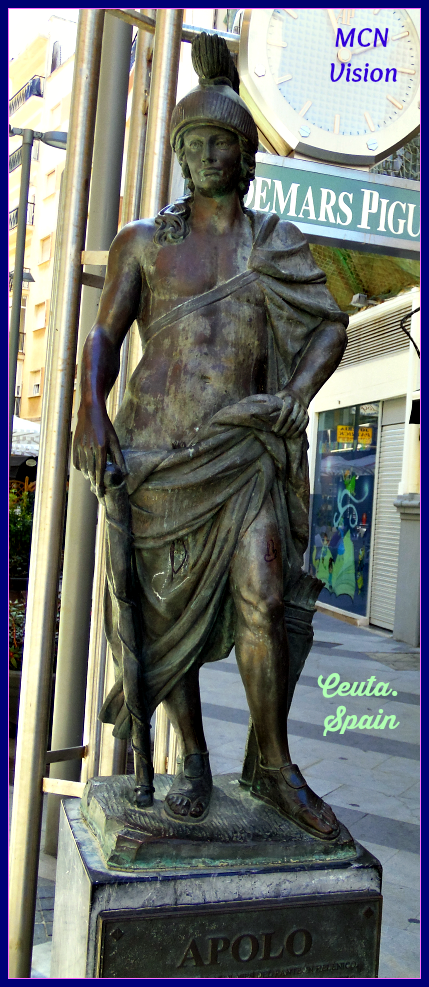The image captures a bronze statue of the Greek god Apollo, prominently displayed in an outdoor marketplace setting in Ceuta, Spain. The statue reveals detailed craftsmanship, with Apollo adorned in a traditional helmet featuring large, flowing plumes extending from the front to the back. His facial features include a well-defined beard, and he's depicted shirtless with a draped tunic or sash that winds around his chest and over one shoulder, while another sash covers his lower body. On his feet, Apollo is wearing sandals, and in his right hand, he holds a cane. The statue is mounted on a square-shaped platform with the name "APOLLO" engraved prominently in capital letters. The platform appears aged, covered in gray dust and dirt. Background elements include a clock overhead and several shop structures, with a light green cursive sign reading "CEUTA SPAIN" to the right. The bronze statue itself exhibits a greenish tint, hinting at its age and exposure to the elements.